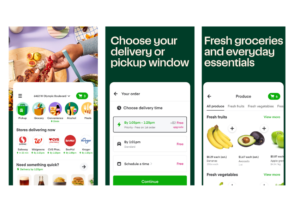The image collage features three phone screenshot images, each providing a glimpse into a delivery or pickup service app, likely from Publix.

In the first screenshot, the top portion shows a plate of food with someone reaching to grab an item off it. Below this, there are five circles, each containing a different image, though the details are too small to discern clearly. Under the circles, there is a title that is not legible, followed by another section showcasing five more images, each representing well-known companies such as Walgreens, accompanied by another title that remains unreadable. Below this are images of a cheeseburger and a wine glass.

The second screenshot is set against a dark green background. At the top, it says "Choose your delivery or pickup window" with a white rectangular box beneath it displaying a back arrow, the text "your order," and "choose delivery time," although the specific times are too small to read. There are two more options below, with the final one switching to red lettering, and a green button at the bottom, presumably labeled "Continue."

The third screenshot, also against a dark green background, prominently displays the message "Fresh groceries and essentials every day" alongside various grocery images.